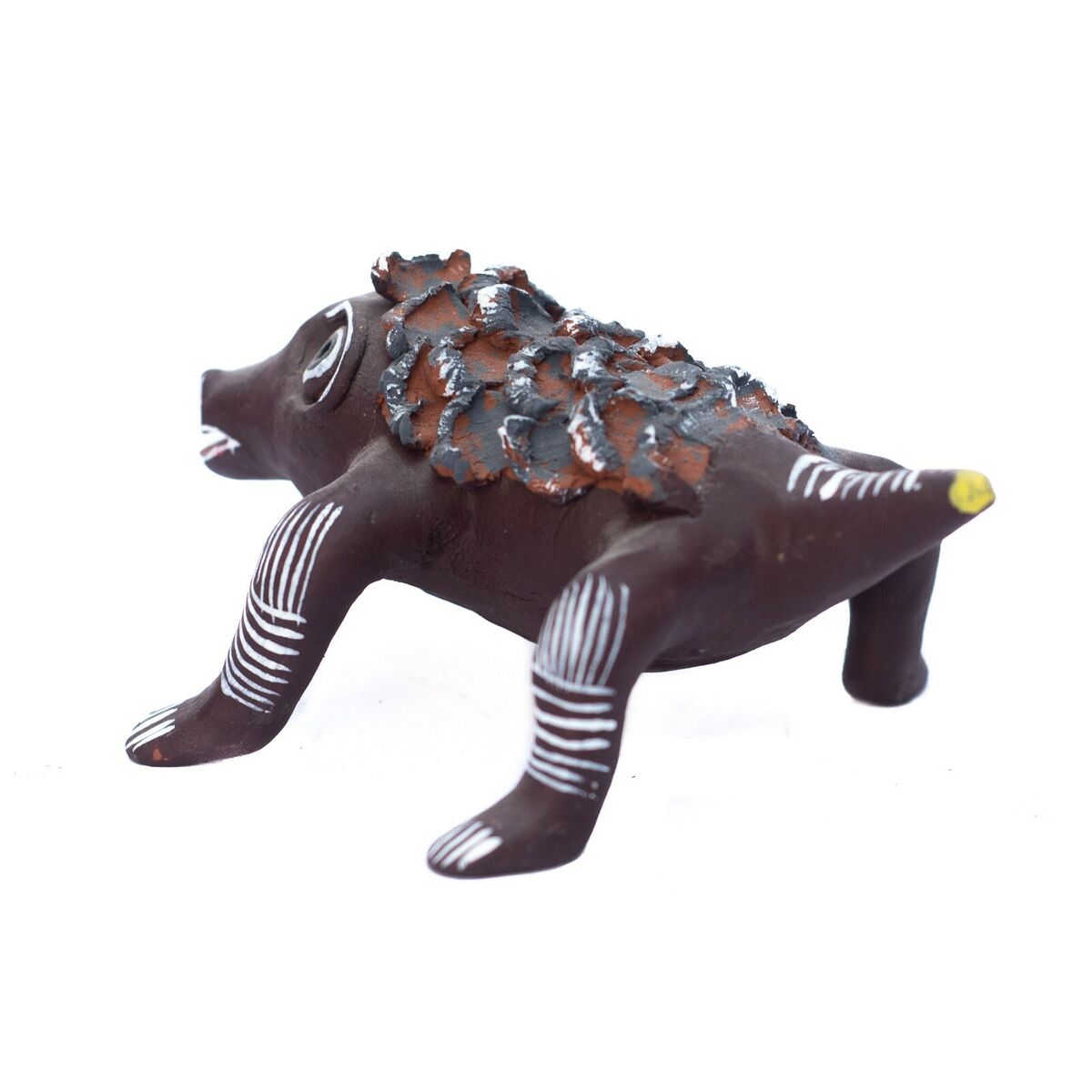This image depicts a handmade clay sculpture of an animal resembling a lizard or armadillo, characterized by a detailed and textured appearance. The creature, primarily rendered in a dark maroon-brown color, is positioned on all fours, with three visible legs featuring carefully painted white stripes along their lengths. The fourth leg is out of view. Each leg also highlights defined white lines, mimicking claws or toes. The tail, short with a yellow dot at its fractured end, showcases horizontal white stripes.

The back of the animal is adorned with scale-like shapes, starting in light brown and transitioning to gray with white tips, emulating a rough, armored texture. This suggests a biological armor or scales. The creature's head is slightly turned, revealing one eye, which is large and expresses a gaze directed upwards. The snout is pointy with a slightly open mouth, marked with white lines around eyebrows, eyes, and mouth, hinting at facial features and perhaps a nose.

Overall, the sculpture appears to be an ancient artifact, possibly photographed for a museum collection, exhibiting a sense of curiosity and lifelike detail despite its rough, handmade construction.